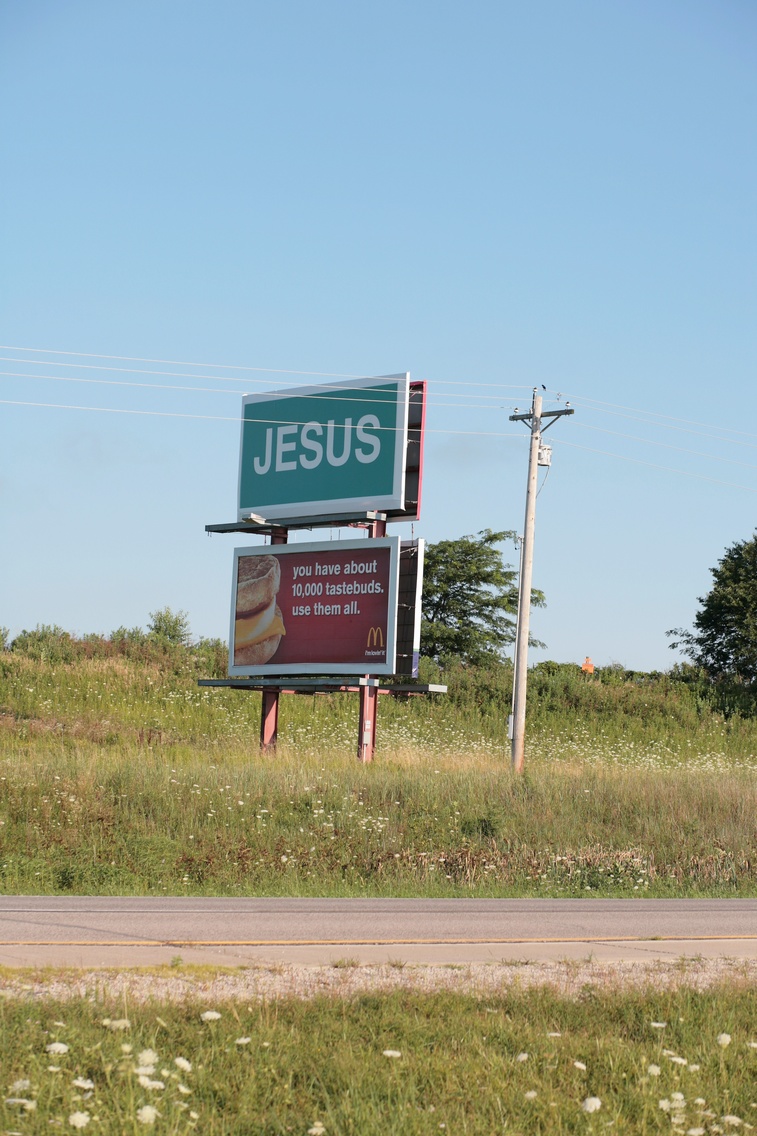This outdoor photograph captures a clear, blue sky without a trace of clouds, providing a serene backdrop for a rural road or highway. Flanking the road, there are patches of green grass interspersed with wild, flowering weeds, suggesting an untamed and natural environment. Dominating the scene is a two-tiered billboard. The top tier features a simple design with a white border and a green center, emblazoned with the word "Jesus" in bold white letters. The bottom tier is an advertisement for McDonald's, characterized by a vibrant red background. It displays an appetizing image of an Egg McMuffin, accompanied by the text, "You have about 10,000 taste buds. Use them all." The iconic golden arches of McDonald’s logo embellish the bottom of the ad.

Behind this prominent billboard, a utility pole with several power lines stretches upwards, adding a touch of industrial complexity to the rural setting. In the background, a few trees stand tall, their leaves adding depth and a touch of greenery to the scene. A small, indistinguishable yellow object is partially visible behind the utility pole; it might be a street sign or another marker, though its identity remains unclear from the image. This captures a moment of juxtaposition between commercial messaging and natural surroundings, creating a visually intriguing landscape.